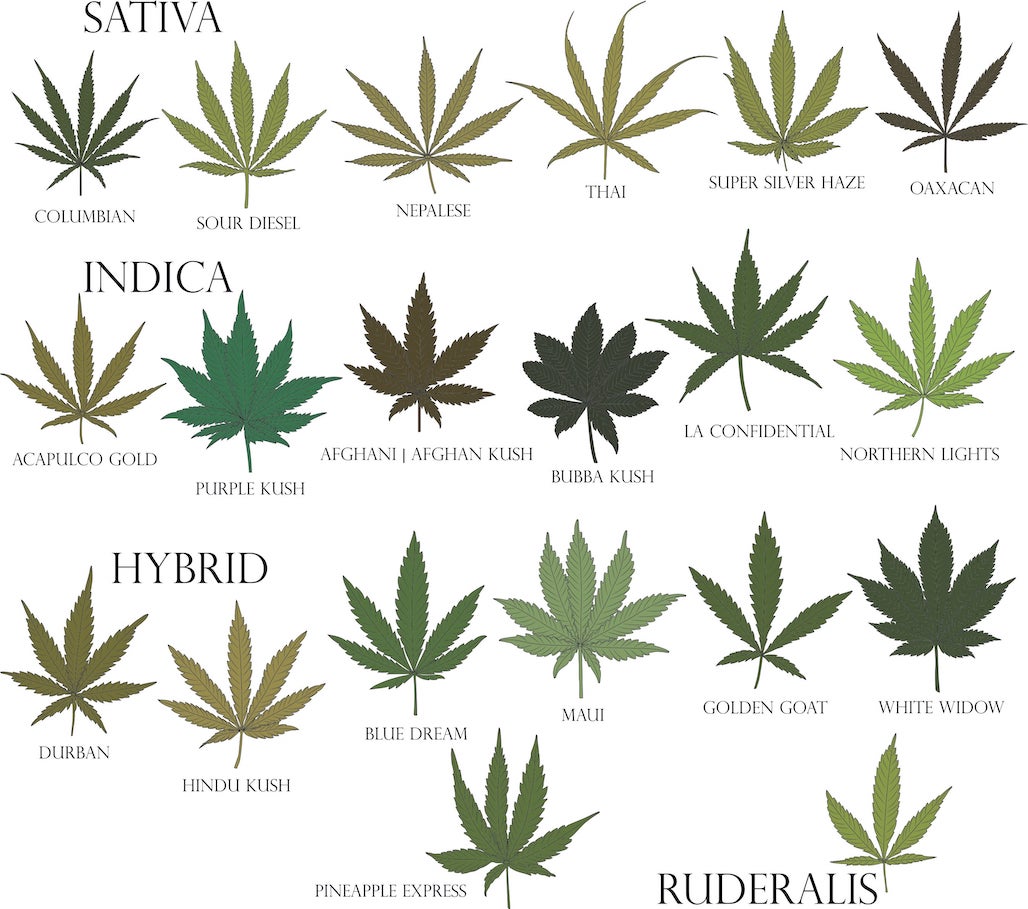The image displays a white background featuring an organized collection of marijuana leaves categorized into four rows. Each row is clearly labeled in black text on the left-hand side, starting with "Sativa" in the first row, which includes leaves named Colombian, Sour Diesel, Nepalese, Thai, Super Silver Haze, and Oaxacan. The leaves vary in shades of green and have different leaf counts, ranging from six to nine. The second row, labeled "Indica," features leaves named Acapulco Gold, Purple Kush, Afghani, Afghani Kush, Bubba Kush, LA Confidential, and Northern Lights. The third row labeled "Hybrid" contains leaves named Durban, Hindu Kush, Blue Dream, Maui, Golden Goat, and White Widow. Finally, at the bottom, there is a single leaf with the label "Pineapple Express" next to the text "Ruderalis". The leaves exhibit a variety of green and brown hues, meticulously arranged to highlight the diversity within each category.